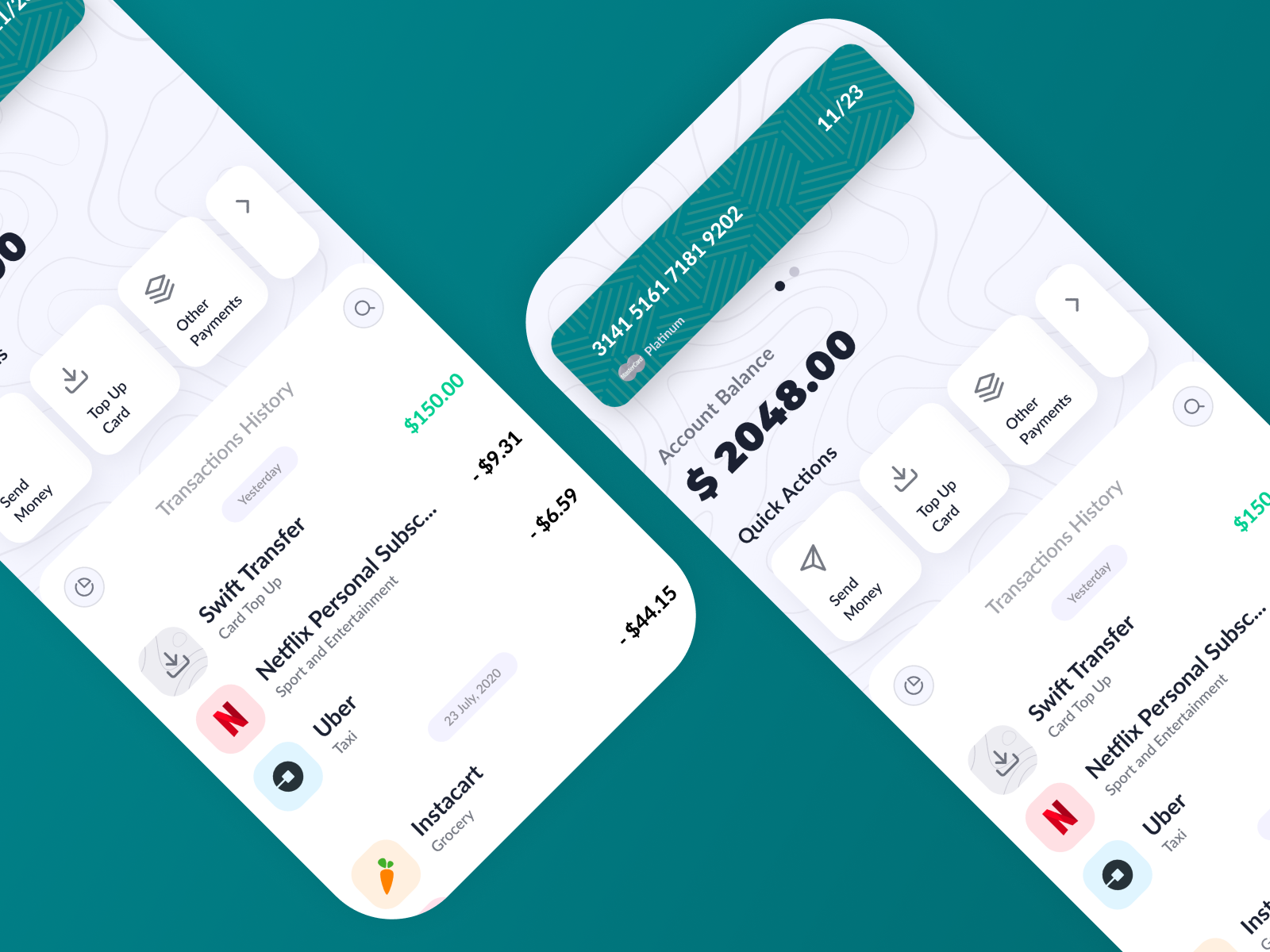In the displayed image, we see a mobile application interface set against a teal backdrop, featuring two phones shown at an angle. The main screen has a gradient gray background with several white boxes containing options in black font. The first white box is labeled "Send Money," and the second box reads "Top Up Card." The third box says "Other Payments," accompanied by a right-facing gray arrow.

Below these options, there's a circular icon with a semicircle inside, labeled "Transaction History" to its right. Adjacent to it is a circle on a gray background featuring a magnifying glass icon. Following this, another gray circle contains the word "Yesterday." To the right of the "Yesterday" icon, texts appear specifying "Swift Transfer, Card Top Up" with a download button on the left. A bright green "$150" figure is also displayed prominently. Beneath this, the Netflix logo, marked by a red "N" within a pink circle, is visible. Next to it, the description reads "Netflix Personal Subscribe Sport and Entertainment," showing a transaction of "-$9.31" in black font.

Further below, a blue circle with a black interior states "Uber Taxi," with a "-$6.59" figure to its right. This is followed by a gray square denoting the date "July 23, 2020." Toward the bottom left is a light brown square with an orange carrot and two green leaves, labeled "Instacart Grocery," and listing a transaction of "-$44.15."

The second phone screen appears with a darker green tint and gray lines. Displayed prominently in white font across the screen is a sequence of numbers: "3141516171819202." On the right of this number sequence, it says "11/23," alongside the MasterCard logo with the designation "Platinum." Below this, there are small black and gray dots, and text reading "Account Balance" followed by "$2048" in black font. Further down, it reads "Quick Actions," with white boxes labeled "Send Money," "Top Up Card," and "Other Payments." An accompanying gray arrow is on the third box, similar to the layout on the first phone screen, concluding with options for "Transaction History" like on the previous screen.